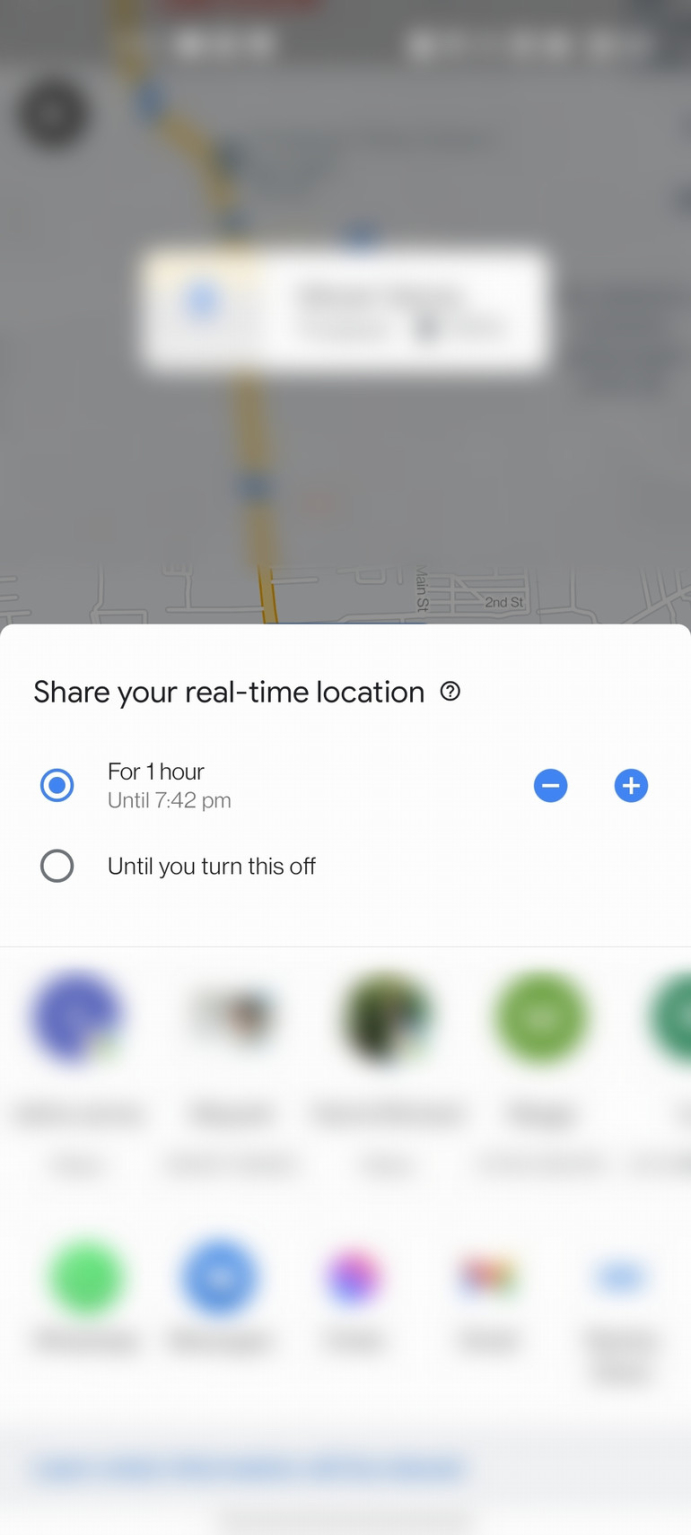The image is a blurred screenshot from a mobile device, characterized by white text at the top center and right. In the middle, there is a partially obscured map in a square format showcasing a yellow highway or roadway running from bottom to top, accompanied by blue highway markers. The top left corner features a black dot or circle, likely a directional button. A pop-up message, also blurred, appears, suggesting options to share your real-time location and offering a blue button to do so for one hour—specifically until 7:42 p.m. Additional interface elements include a question mark button, as well as plus and minus icons. The pop-up also has a blank section after the text "until you turn this off." At the bottom of the screen, several application icons are visible but blurred, displaying a range of colors—green, blue, pink, purple, red, and yellow—arranged in circular shapes, indicative of various apps.